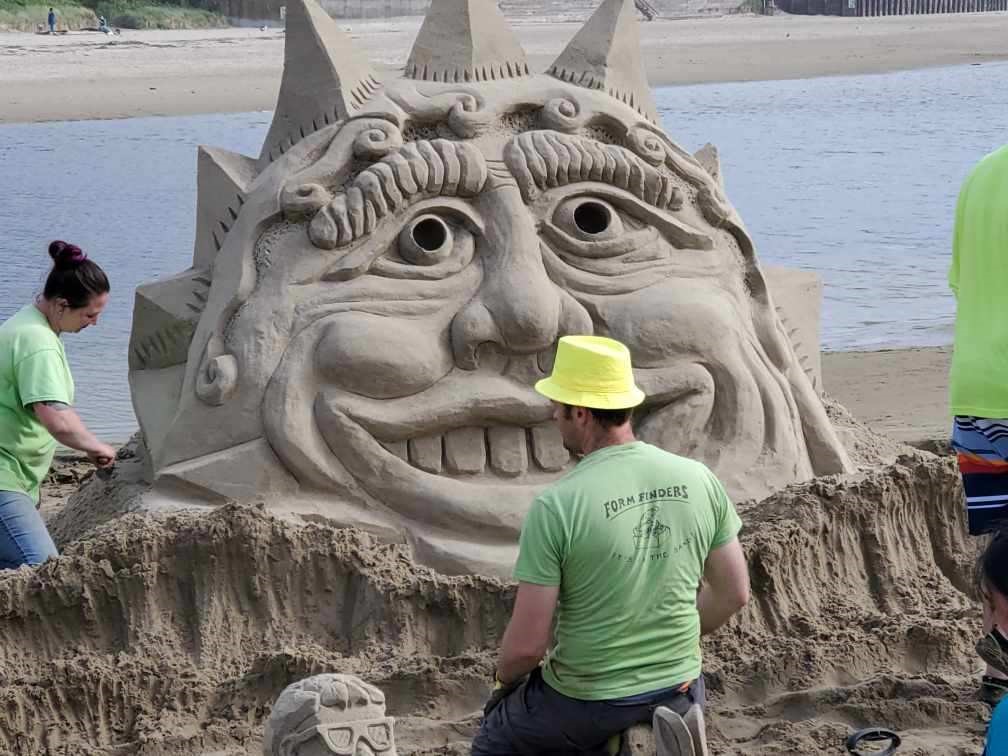In this detailed color photograph taken at the beach, a monumental sand sculpture captures immediate attention. The main focal point is an incredibly elaborate figure reminiscent of a king with a prominent crown perched on his head. The craftsmanship of this sandy monarch is astonishing, featuring a smiling face complete with expressive and lumpy cheeks, large lips, and pronounced teeth. The king’s detailed countenance is filled with character, with carefully sculpted eyes and nose.

Nestled at the bottom left corner of this intricate artwork is a smaller face, notably unexpressive, but adorned with sunglasses and some hair, adding a whimsical touch to the scene. Surrounding this sand masterpiece, three individuals are partially visible, all wearing neon light green t-shirts emblazoned with the words "Form Finders." These artists are diligently sculpting the sand, contributing to the stunning creation that boasts a backdrop of a tranquil water lagoon and expansive beach.

Interestingly, one might observe that the main sculpture shares a striking resemblance to the transformed monster head of Chet from the classic film "Weird Science," particularly recognizable by its detailed and expressive monstrous features. This engaging scene not only showcases impressive artistry but also transforms a simple day at the beach into a showcase of creativity and skill.